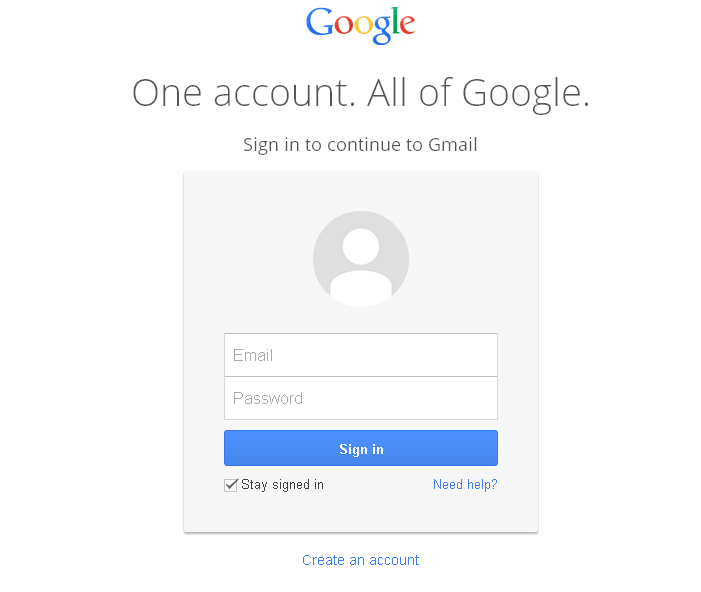This is a colored image showcasing a Google sign-in screen, set against a white background. Dominating the center of the image is the iconic Google multi-colored logo, with each letter distinctly colored: 'G' in blue, 'o' in red, 'o' in yellow, 'g' in blue, 'l' in green, and 'e' in red. Below the logo, dark grey text reads: “One account. All of Google. Sign in to continue to Gmail.”

The sign-in section features a slightly grey background within a squarish outline. There is a faint grey line at the bottom of this square, and possibly very thin lines on the left and right sides. Central to this section is a round icon depicting a grey head and shoulders silhouette.

Below this icon are input boxes for email and password, followed by a blue rectangular 'Sign in' button with white text on it. Below the 'Sign in' button, to the left, there is a checkbox labeled "Stay signed in," which is ticked and written in black. On the right side, blue text reads, “Need help?”

At the bottom of this section, centered within the image, there is more blue text reading, "Create an account." The overall composition suggests this image was likely captured from a website or possibly a mobile device screen, focusing solely on the Google sign-in interface.